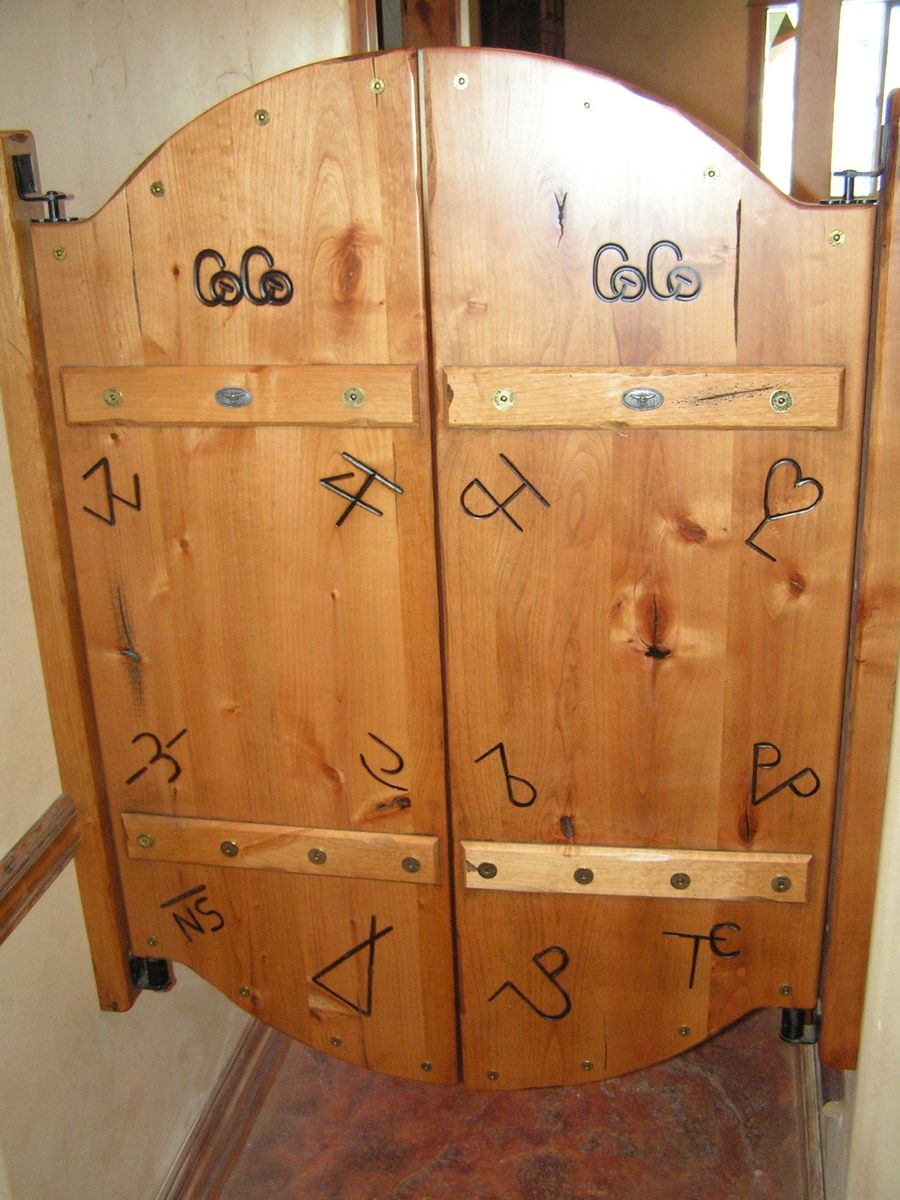The photograph showcases a pair of wooden swing doors resembling classic saloon doors. These double doors are crafted from wooden material with a smooth, well-polished brown surface and feature elegant black hinges on both sides. The doors are defined by an arch at both the top and bottom.

Intricate carvings adorn the front of the doors, with some inscriptions reading "cocoa" and motifs such as hearts, alongside more abstract and unidentifiable patterns. These carvings are highlighted in black, suggesting they were etched using a sharp implement.

The floor beneath the doors appears aged and is a reddish hue, likely constructed from concrete or natural rock. The surrounding environment includes a cream-colored wall to the left, with additional walls and a door visible in the background. The picture was taken with a flash, creating a notable highlight on the wooden surface, accentuating the door’s polished finish.